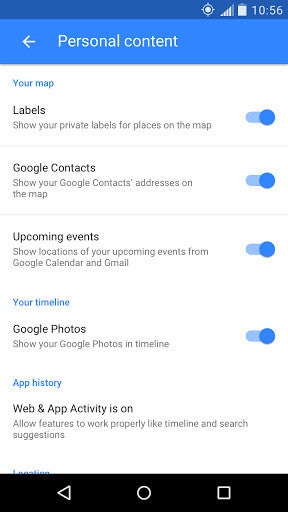This is a detailed screenshot from an Android phone's "Personal Content" section within the settings menu. 

At the top, the status bar displays the time as 10:56, a nearly full battery icon, and four out of five bars for cellular signal strength.

Below the status bar, a blue header labeled "Personal Content" is accompanied by a left-pointing arrow to navigate back in the menu.

The main screen is segmented into various sections with respective statuses:
1. **Labels**: "Show your private labels for places on the map" - this option is enabled.
2. **Google Contacts**: "Show your Google contacts' addresses on the map" - this option is enabled.
3. **Upcoming Events**: "Show locations of your upcoming events from Google Calendar and Gmail" - this option is enabled.
4. **Your Timeline**: "Show your Google Photos and timeline" - this option is enabled.
5. **App History and Web and App Activity**: "Allow features like timeline and search suggestions to work properly" - this option is enabled.

At the bottom of the screen, a black navigation bar hosts three buttons: the Back button, the Home button, and the Recent Apps button for managing open applications.

This screenshot exemplifies the various privacy and display settings available on an Android phone's map-related features.